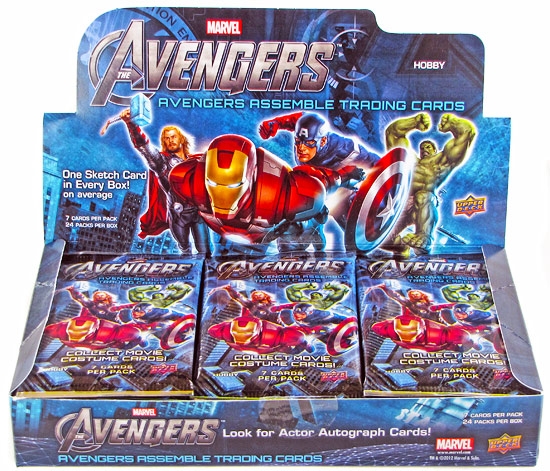This color photograph features an open display box of Marvel's Avengers Assemble trading cards. The box lid displays prominent silver text stating "Avengers," topped by a red box with white text reading "Marvel." Below in blue text, it reads "Avengers Assemble Trading Cards." On the box lid, illustrations of four Marvel superheroes are prominently featured: Thor with his hammer and red cape, Iron Man in his red and gold metal suit, Captain America in his red, white, and blue suit with an 'A' on his forehead, and the Hulk raising his fists angrily. The same imagery is found on the three stacks of wrapped cards inside the box. The box also highlights additional features with white text stating, "One sketch card in every box on average" and "Look for actor autograph cards." The right margin of the box includes the word "Hobby" in white text.